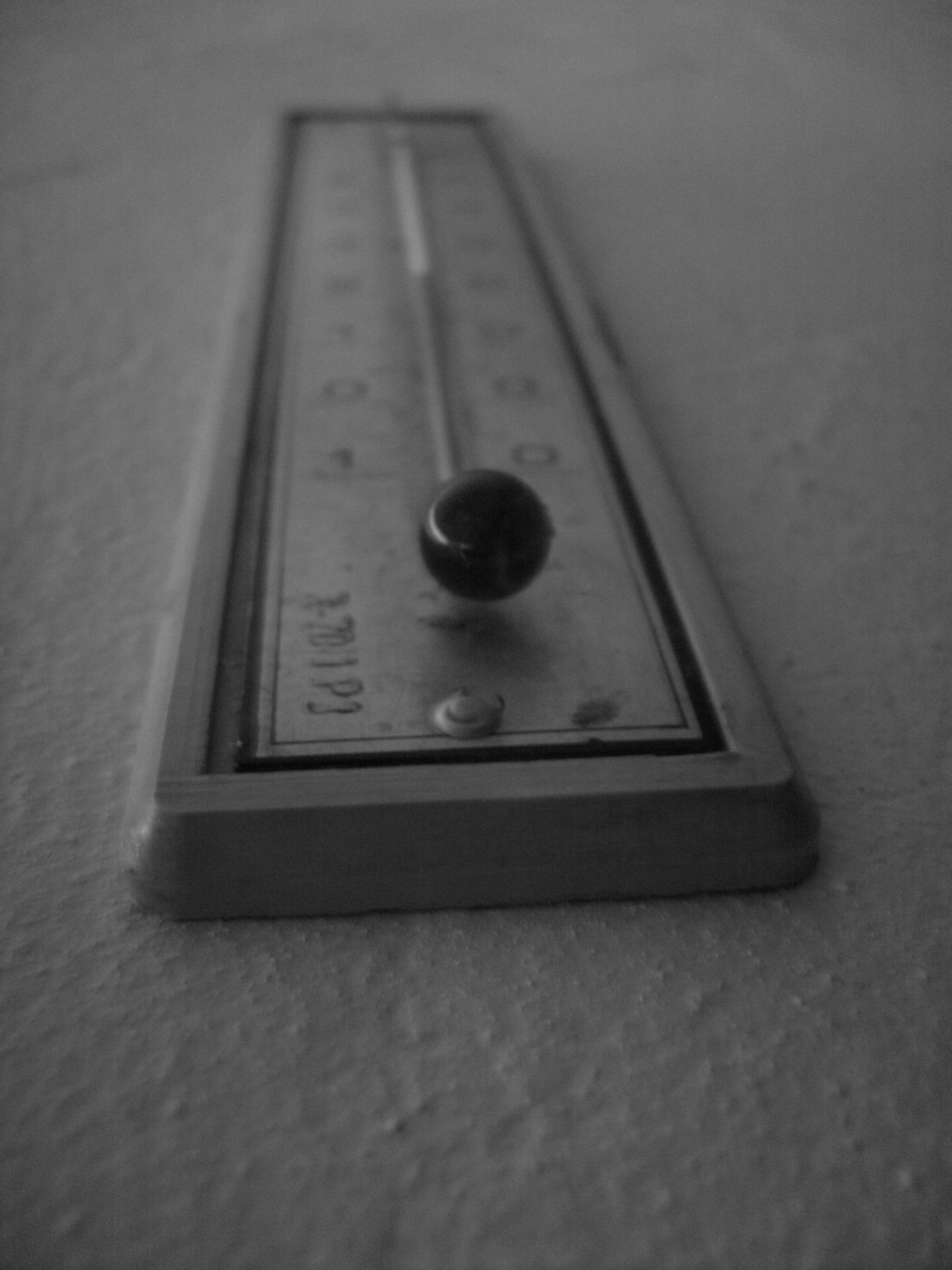This is a detailed black-and-white portrait-style photograph captured from a low angle. The image focuses on a vintage thermometer placed on a rough, light-colored concrete surface. The composition captures the thermometer from the bottom, centered in the frame, and extends towards the top, where the image starts to blur around the halfway point. Dominating the center bottom of the photograph is a large, black bulb, indicative of traditional mercury or spirit thermometers. On the thermometer's scale, there's a small, white, rectangular indicator that is filled with red fluid up to the midpoint, signifying zero degrees. Faint, blurry numbers flank the indicator, with '1' on the left and '0' on the right. The thermometer itself is encased in a rectangular metal frame with rounded corners, adding a classic touch to the image.